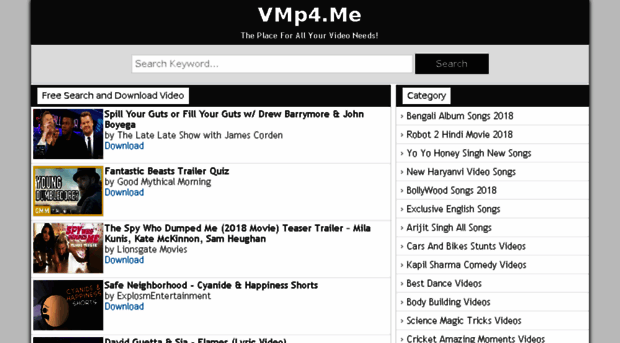The image showcases a video platform interface with the header "VMp4.ME" displayed prominently at the top in a mix of capital and lowercase letters. The tagline "The place for all your video needs!" is boldly presented against a black background. The left and right sides of the image feature a light gray background.

Centered beneath the tagline is a search bar labeled "Search keyword," flanked by a black search button set against a light gray background. Below the search bar, it says "Free search and download videos," followed by the word "Category" with a small white rectangle next to it.

On the left side of the image, there are four video thumbnails, each accompanied by their respective titles in black text:
1. "Spill Your Guts or Fill Your Guts with Drew Barrymore and John Boyega"
2. "Fantastic Beasts Trailer Quiz"
3. "The Spy Who Dumped Me 2018 Movie Teaser Trailer" featuring Mila Kunis, Kate McKinnon, and Sam Heughan
4. "Safe Neighborhood" from Cyanide & Happiness Shorts

To the right, under the "Category" section, a list of 13 clickable categories is displayed in gray text, allowing users to navigate through the various video content available on the platform.